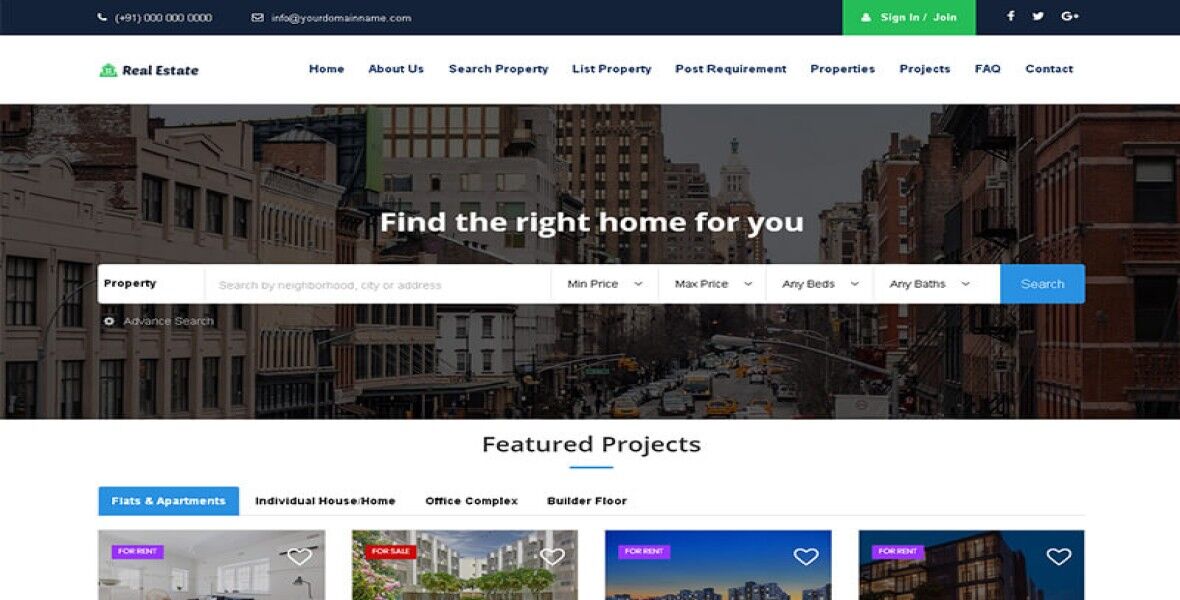This is a screenshot from a real estate website. At the top, there is a navy blue bar displaying a phone number with a country code starting with +911. This bar appears to be part of a template featuring an email address formatted as info@yourdomainname.com. On the right side of the page, there is a green button labeled "Sign In/Join," accompanied by icons for Facebook, Twitter, and Google Plus. Below this, a white bar prominently displays the name of the website “Real Estate,” along with several navigation tabs: Home, About Us, Search Property, List Property, Post Requirement, Properties, Projects, FAQ, and Contact.

The background of the page features a grayed-out image of New York City, overlaid with the text "Find the right home for you" in large white letters. Beneath this text is a search bar allowing users to search for properties by neighborhood, city, or address. This bar includes dropdown menus for minimum price, maximum price, number of bedrooms, and number of bathrooms, followed by a blue "Search" button.

Further down, the page highlights "Featured Projects," providing categories for users to browse through: Flats and Apartments (which is currently selected and highlighted in blue), Individual House/Home, Office Complex, and Builder Floor. Several images of properties available for sale or rent are shown, although only partially visible in the screenshot.